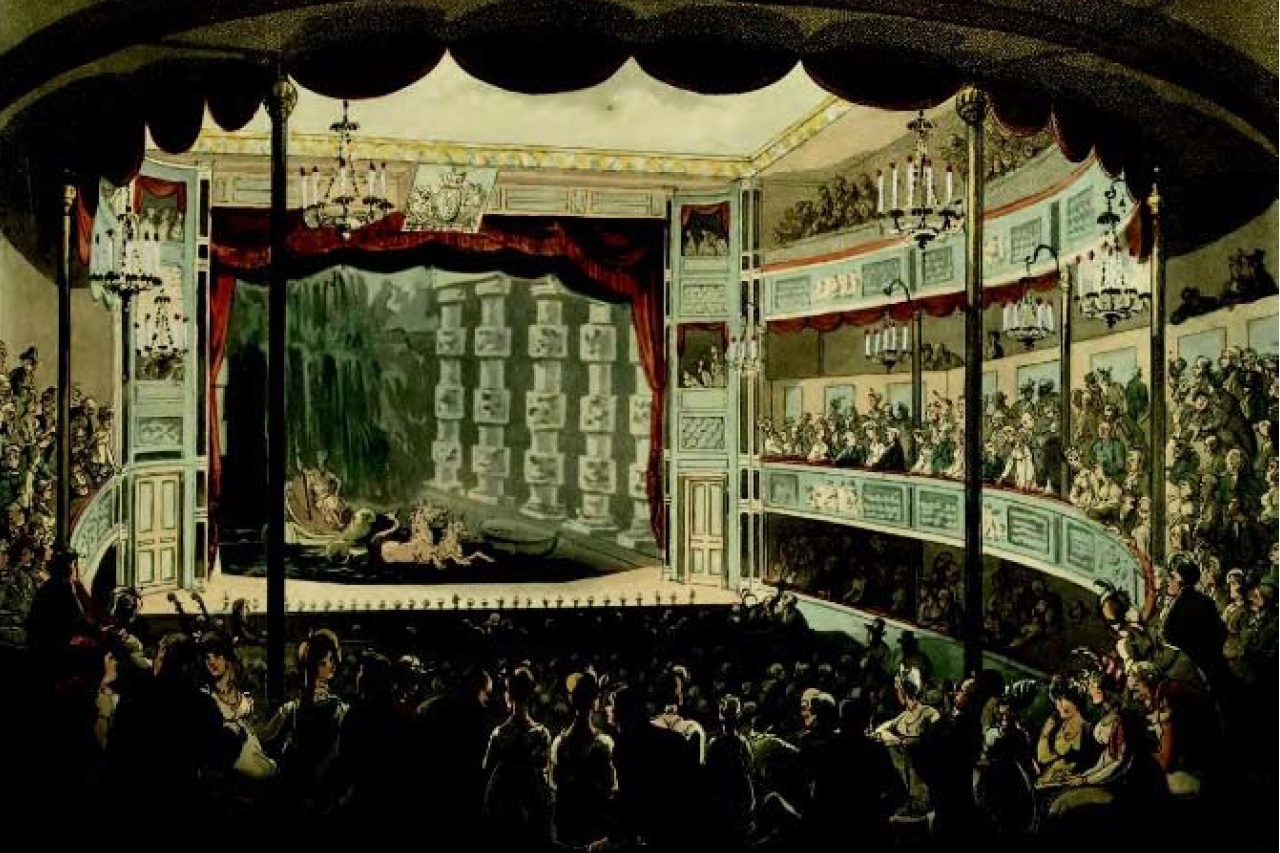This detailed painting depicts a lavish theater interior evocative of the 1700s or 1800s, filled with an audience dressed in period attire. The theater is circular in shape, featuring multiple levels of seating, including balconies, a floor level, and a loge section, which is filled with men and women seated and observing the stage. The stage itself is ornate and prominently features a red curtain at the top, with a chandelier hanging from the ceiling. The backdrop of the stage consists of a green, forest-like scene with columns drawn on a screen, suggesting an outdoor setting.

In the center of the stage, there is a carriage or cart being drawn by two animals, which upon closer inspection appear to be either horses or large dogs like Great Danes, and inside the carriage, a woman character is seated. The overall lighting of the painting is provided by chandeliers with candle-like fixtures hanging from the theater's ceiling, casting a warm glow over the scene. The right side of the theater reveals additional balconies filled with spectators, providing a lively and immersive atmosphere to this richly detailed and historic setting.